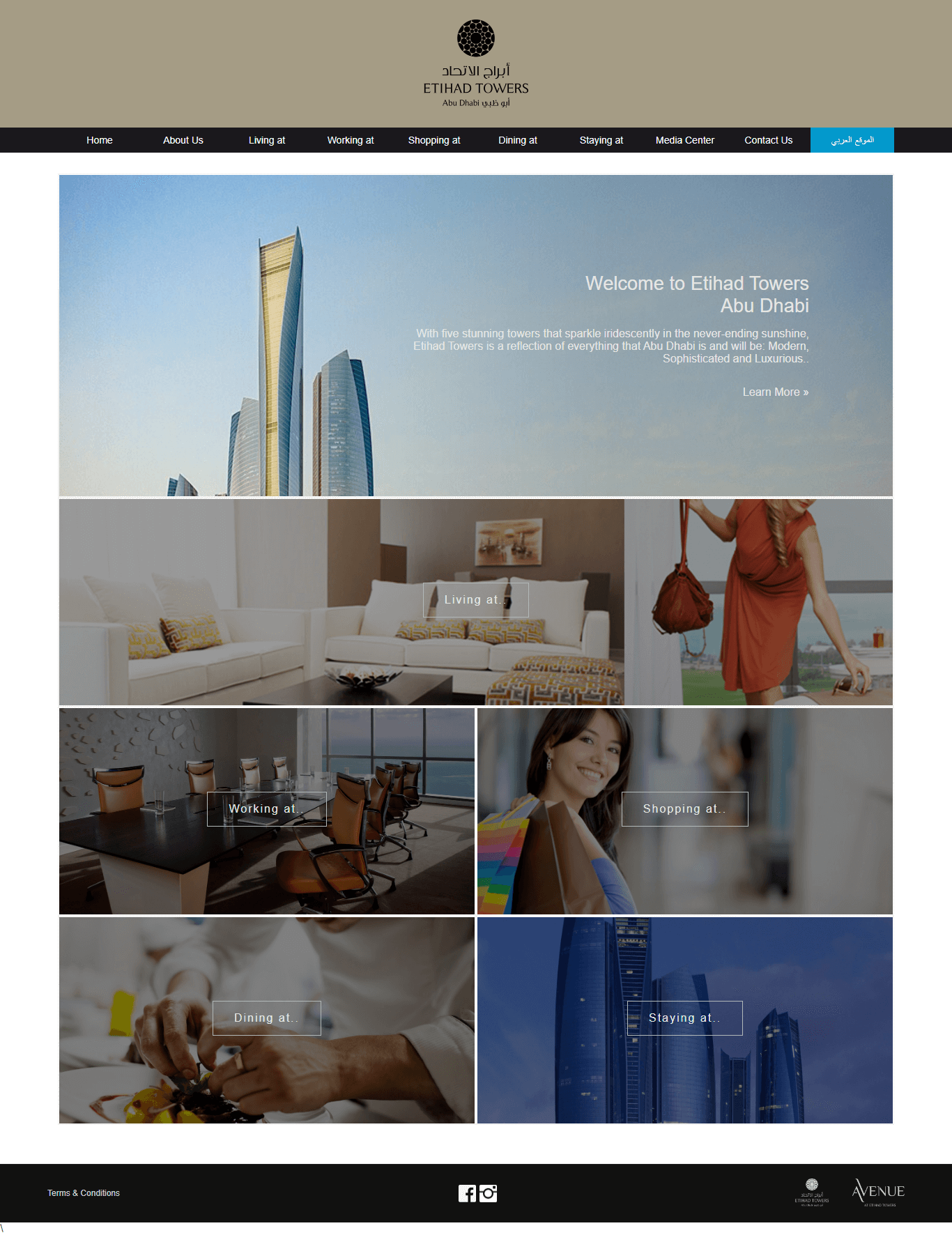Website for Ediad Towers in Abu Dhabi

At the top of the website, a beautifully designed header features the name "Ediad Towers" prominently in elegant script, beneath which "Abu Dhabi" is inscribed, possibly in Farsi, adding a touch of cultural authenticity. 

Navigation options are seamlessly integrated within the header, allowing users to effortlessly explore sections such as: Home, About, Living, Working, Shopping, Dining, Staying, Media Center, and Contact Us.

The main section below the header welcomes visitors with a captivating photograph of the Ediad Towers in Abu Dhabi, described as two stunning towers that dazzle in the perpetual sunshine. The description emphasizes Ediad Towers as a quintessential emblem of Abu Dhabi's modern, sophisticated, and luxurious aspirations. A 'Learn More' button invites users to delve deeper into what Ediad Towers has to offer.

Further down, the "Living" section showcases a collection of house and domestic products, including furniture and artwork designed to complement modern living spaces. The imagery features a woman on the left, stylishly grabbing her purse and sunglasses, seemingly ready for a shopping venture.

Adjacent images highlight different aspects of the Towers. The "Working" section displays sleek office furniture, including a sharp-looking black table with a white base, surrounded by brown leather chairs accented with black metal frames. 

On the right, the "Shopping" section features an image of a woman carrying two shopping bags, embodying the upscale retail experience that Ediad Towers promises.

Adjacent to this, the "Dining" section captures a chef intricately preparing a gourmet plate, hinting at the fine dining experiences available. To the right, a striking image showcases the five towers of Ediad, standing tall against the Abu Dhabi skyline, solidifying the grandeur and architectural elegance of the Ediad Towers.

This detailed layout ensures visitors are treated to an immersive preview of the luxurious and multifaceted lifestyle that Ediad Towers aims to provide.